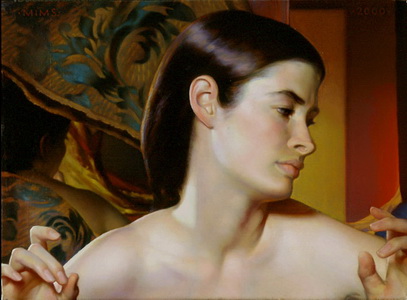The image is a realistic painting, almost photographic in detail, of a young, light-skinned woman in her 20s. Her long dark brown hair is pulled back behind her ears and held out of view behind her neck and back. The focus is on her head and shoulders, leaving it ambiguous whether she is wearing a strapless dress or is otherwise unclothed from the shoulders down. She is depicted looking downward over her left shoulder with a thoughtful expression.

Her hands are posed near her shoulders: her right hand forms an 'OK' gesture, with the middle finger touching the thumb and the other fingers curved back. In contrast, her left hand is open, with fingers slightly spread, and her palm facing inward towards her body. These delicate hand gestures add a layer of grace to her portrayal.

The backdrop features a combination of blue and green floral patterns on a golden fabric to the left, and a tapestry-like arrangement with gold and orange horizontal elements on the right, adding a rich, textured context to the scene. The indoor setting is further defined by the contrast between the soft draped silk on one side and the boxy, vibrant red and yellow background on the other.